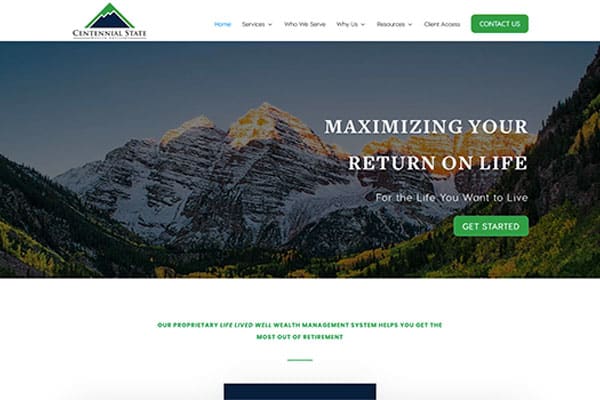The website homepage for Centennial State presents a comprehensive user interface designed for a seamless navigation experience. On the right side of the main page, there is a region featuring several navigation options including a "Home" button, a blue "Services" dropdown menu, and submenu links titled "Who We Serve" and "Why Us." Additionally, there is a "Resources" button and a "Client Access" link. To the far right, a green "Contact Us" button is available for users who need to get in touch with the team for further assistance.

Below this navigation menu features a stunning image of a natural landscape, showcasing a series of rocky mountains characterized by distinct white horizontal striations. The image captures sunlight filtering through the mountain peaks, illuminating a gentle sloping valley dotted with trees on the left and right sides.

Beneath this scenic photograph, in small green capitalized text, is a motivational phrase, "OUR PROPRIETY LIFE LIVE WELL WEALTH MANAGEMENT SYSTEM," which emphasizes the website's focus on retirement planning and financial management.

Further down, a thin green line precedes a large, dark blue (or black) horizontal block, reinforcing the site's financial expertise. The footer reiterates the key navigation options, including access to various services, an "About Us" section, and a "Contact" option for further inquiries, emphasizing Centennial State's commitment to aiding in financial and retirement planning.